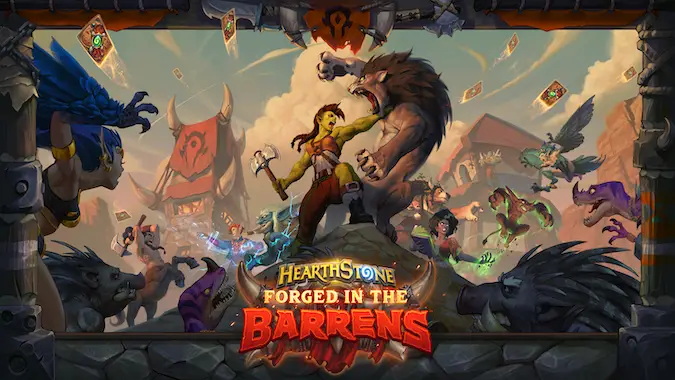The image appears to be a promotional illustration for a video game, specifically for a patch or expansion called "Hearthstone: Forged in the Barrens." The central character is a green-skinned, muscular orc-like creature with braided hair and a mohawk, brandishing an axe and seemingly engaged in combat with a large lion-like werewolf. Surrounding them, the scene is chaotic and vibrant, teeming with various fantasy creatures including elf-like beings, centaurs, dinosaurs, and bird-like females with human torsos. Additional fantastical elements include electrical creatures, flying cards, and numerous other characters in a vibrant, animated or computer-generated style. In the background, there are huts adorned with large horns and clouds, lending to the fantastical setting. The border of the image has a wooden and stone design, and prominently displayed at the bottom of the image is the logo "Hearthstone: Forged in the Barrens" with "Barrens" in large, raised reddish-orange text and "forged in" in fiery orange letters.